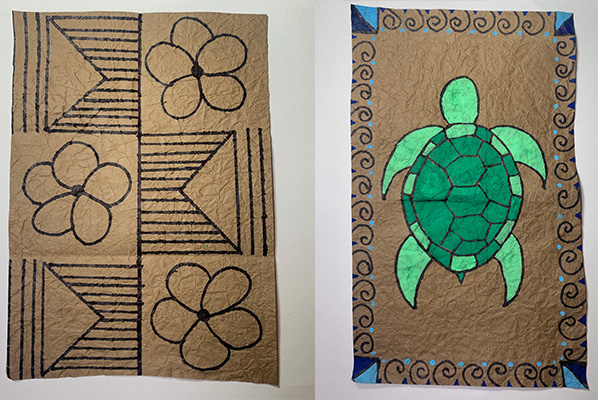This image features two side-by-side color photographs of artwork, each depicted on brown paper with distinct but complementary designs. The photograph on the left displays a detailed ink drawing of flowers and various geometric patterns. Specifically, it showcases three rows with alternating floral and stripe-embellished envelope-like symbols, arranged with two patterns in each row. The flowers, composed of swirling black lines, are positioned thoughtfully across the composition—two in the corners and one centrally placed.

The right photograph highlights a meticulously drawn image of a green sea turtle positioned in the center. The turtle is framed by an intricate border featuring black spirals and dual-colored blue triangles marking the corners, blending light and dark blue hues. Both pieces exhibit a balance of natural and geometric elements rendered in a representational realism style, emphasizing the harmony between organic forms and structured patterns. The overall positioning of the photographs creates a cohesive landscape orientation, further unifying the two different yet harmonious artworks.